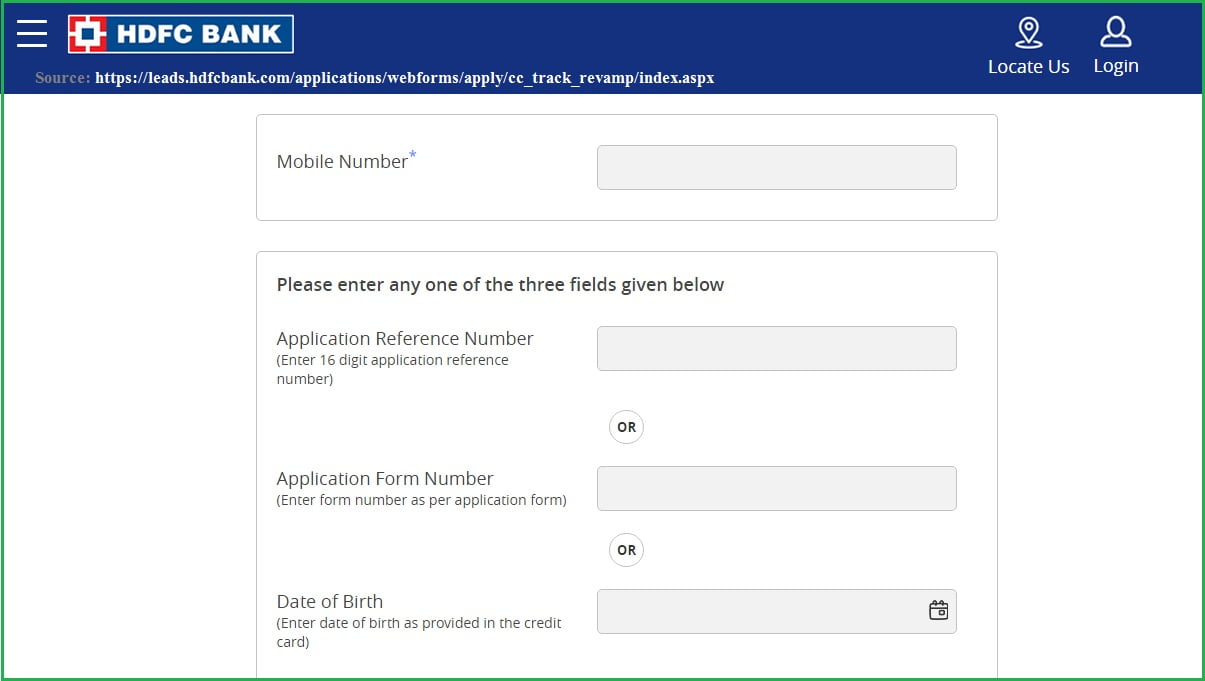The image is a screenshot taken from a web page of the HDFC Bank website. At the top of the screenshot, there is a navigation bar with a blue background. On the left side of this bar, there is the HDFC Bank logo, followed by three horizontal white lines, indicating a menu icon. Next to this, on the right side, there is a small pin icon labeled "Locate Us" and a silhouette of a person labeled "Log In."

Below the navigation bar, the URL of the page is visible, starting with "https://leads.hdfcbank.com," followed by additional slashes and words. The main content area beneath this is predominantly white, except for input rectangles which are gray.

At the top of the content area, there is a prompt asking the user to enter their mobile number. Below this, another prompt instructs the user to "Please enter any one of the three fields given below." These fields are labeled as follows: "Application Reference Number," with a subtext requesting a 16-digit reference number; "Application Form Number"; and "Date of Birth."

The entire image is accented by a bright green border that surrounds it, adding a contrasting frame to the otherwise muted color scheme of the page. The design of the page is clear and structured, guiding users through the necessary steps for form submission or login.